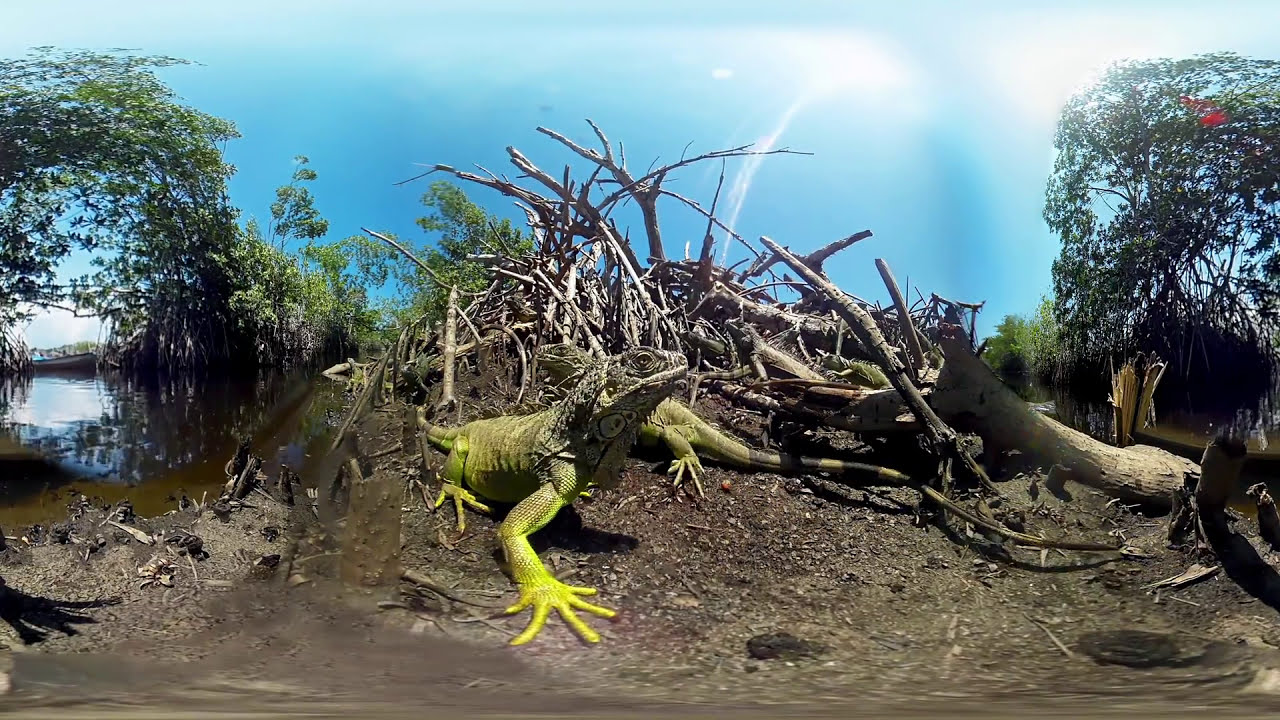The photo captures a vivid outdoor scene featuring two iguanas prominently in the center. Both iguanas, with their rough, flicking faces, exhibit a lighter shade of green across their bodies while their feet stand out in a bright, almost greenish-yellow hue. The iguanas are positioned on a mound of dirt, alongside a pile of dry, tangled branches and debris, possibly resembling a beaver dam. To the left, a shallow pond extends outward, adding a reflective element to the natural setting. The backdrop showcases a dense line of trees stretching horizontally from left to right, with a bright blue sky overhead indicating it's midday. The sunlight streaming from the top right casts clear shadows, enhancing the textures and details of the lizards and their habitat.